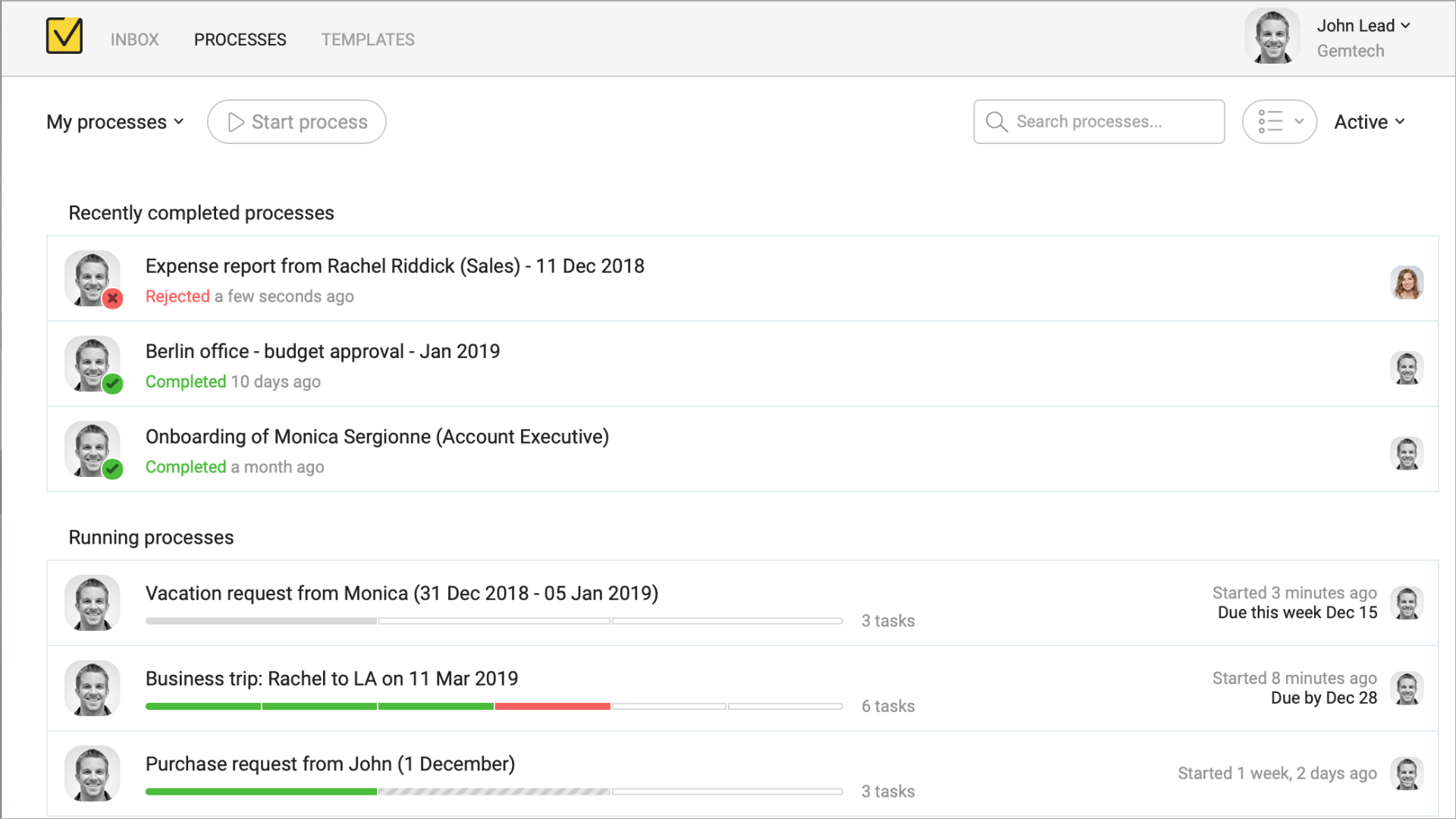In the top left corner of the image, there is a filled yellow square bordered in black. Adjacent to the top right of the yellow square, there is a small opening featuring a black checkmark, with the top part of the checkmark extending near this opening. Moving further to the right, there is light gray, capitalized text that reads "INBOX." To the right of "INBOX," the text "PROCESSES" is capitalized and black, indicating it as the selected section. Next to "PROCESSES," towards the right, there is light gray text that says "TEMPLATES." On the far right side, the bold black name "John Leed" appears, with "GEMTECH" written in smaller gray letters beneath it. An avatar displaying John Leed's grayscale photo is seen to the left of his name.

At the bottom, the image has a white background encapsulating the entire webpage, highlighted by the text "MY PROCESSES" found near the center. In the top left, a black drop-down arrow is visible. To the right of this arrow, there is a long, oval-shaped button outlined in light gray, featuring a play icon and the text "START PROCESS." Adjacent to this button on the right, a search bar reads "SEARCH PROCESSES..." in light gray and is accompanied by a magnifying glass icon. Further to the right of the search bar, there are three lines with bullet points next to them, denoting a drop-down menu with a downward-pointing arrow. Nearby, bold black text that reads "ACTIVE" is followed by a downward-pointing arrowhead. Below this, bold black text states "RECENTLY COMPLETED PROCESSES," under which the first entry showcases the user's avatar and a red X in the bottom right corner.